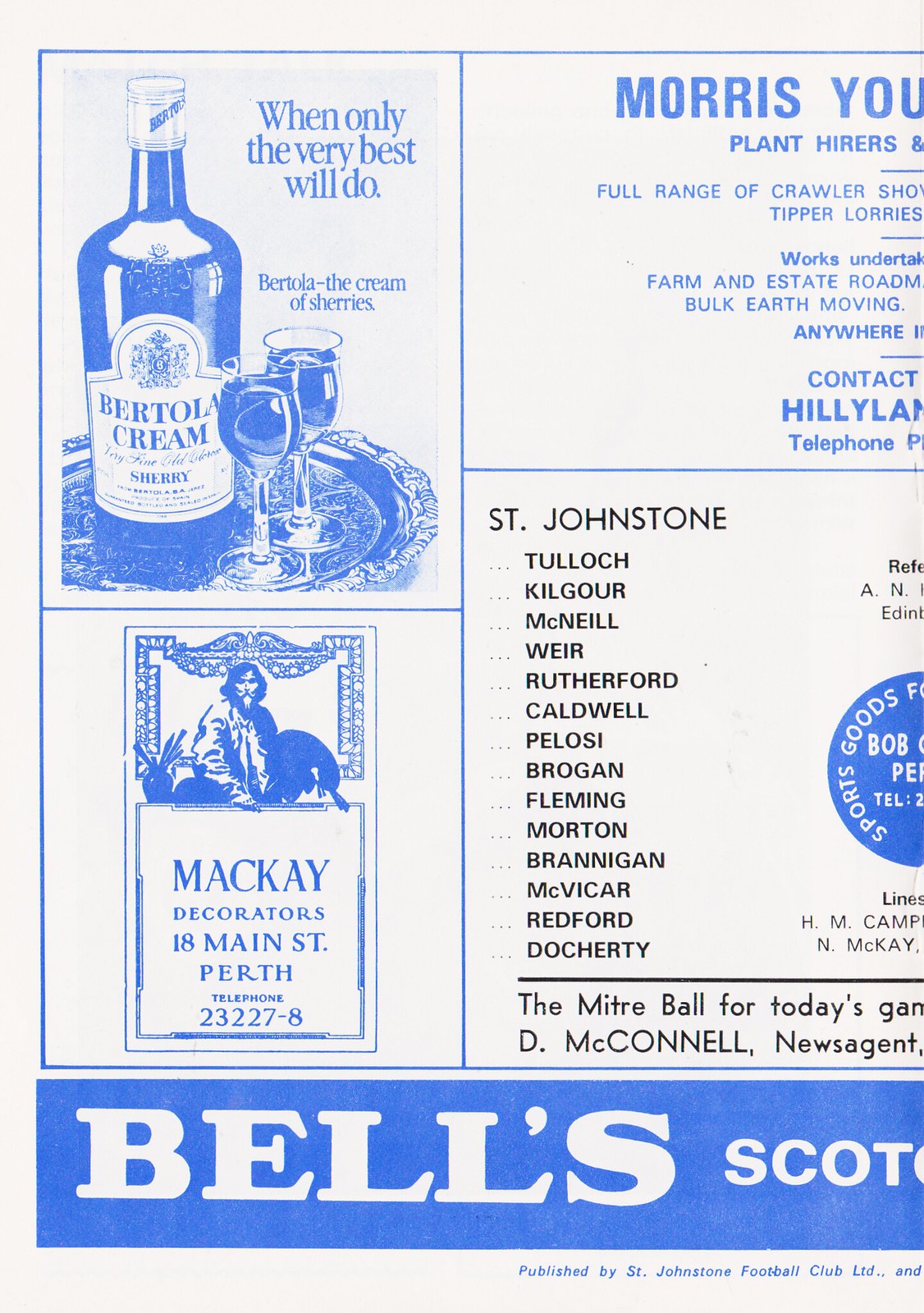The image is a partial advertisement placemat, likely from a restaurant, featuring white with blue text and illustrations, along with some black text. At the upper left corner, there's a monochrome blue illustration of a wine bottle and two glasses on a silver tray, accompanied by the text, "When only the very best will do. Bertola, the cream of Sherry's." Directly below it, there is an advertisement for "Mackay Decorators," located at 18 Main Street, Perth, with a graphic of a man and a telephone number. The upper right section of the image features text for "Morris U," detailing plant hires including crawlers, tippers, and estate equipment, though this section is partially cut off. At the very bottom, a blue rectangle spans across with white letters spelling out "Bell's Scott," though part of this text is also cut off. On the bottom right, there's additional black text for "St. Johnston," followed by a list of names including Tulloch, Kilgore, McNeil, Weir, Rutherford, Caldwell, Pelosi, Brogan, Fleming, Brannigan, McVicar, Redford, and Dougherty.